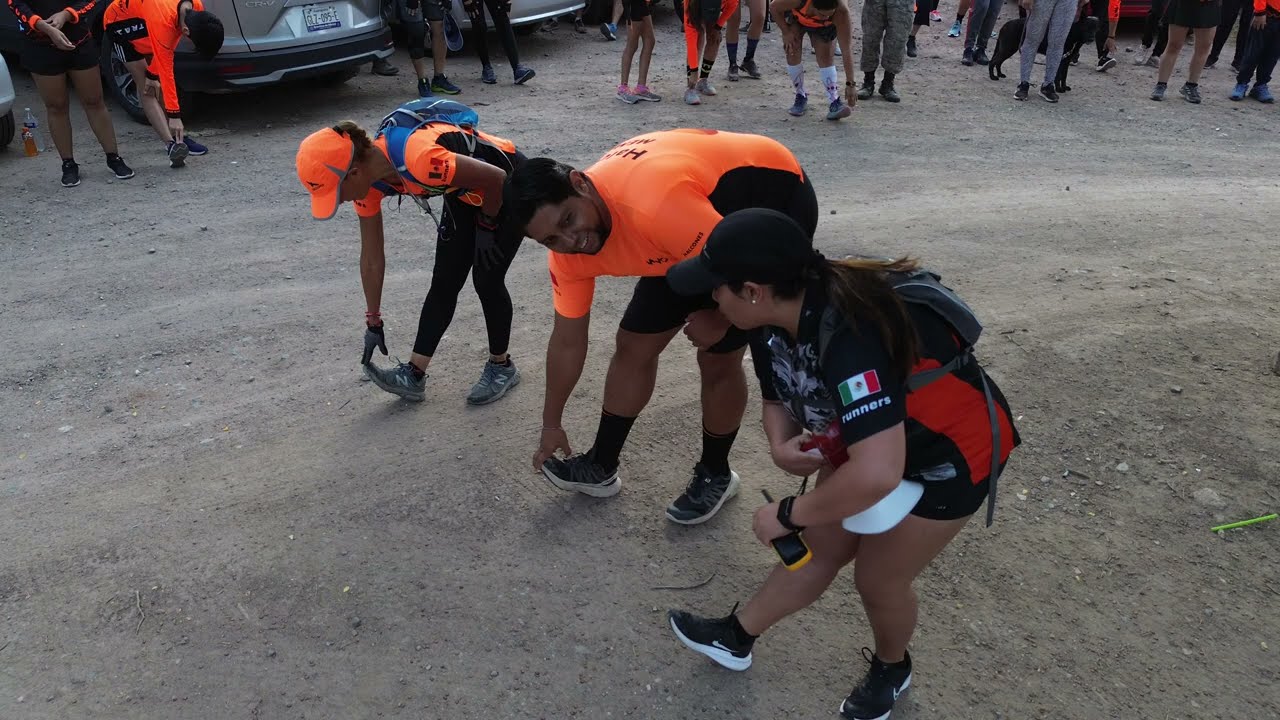In a photograph of a dirt and gravel road, three individuals are captured in mid-stretch, preparing for a marathon or a walking event. Two women flank a man in the center, all appearing to be of Hispanic descent. The man, centered in the frame, wears a distinctive orange and black leotard with short sleeves and knee-length shorts, complemented by black socks and black-and-white shoes. To his right, a woman sports an outfit with long leggings instead of shorts, an orange hat, and a blue backpack, along with gray shoes. She mirrors his stretch. On his left, another woman dons a black and red t-shirt featuring a flag with green, white, and red colors and the word "runners" beneath it. Her ensemble includes black biker shorts, a black cap, and a yellow and black device in her hand, possibly a phone or walkie-talkie, and black-and-white sneakers. The background is alive with activity, showing numerous spectators and participants from the waist down, while vehicles are also visible, signifying the start of the race.